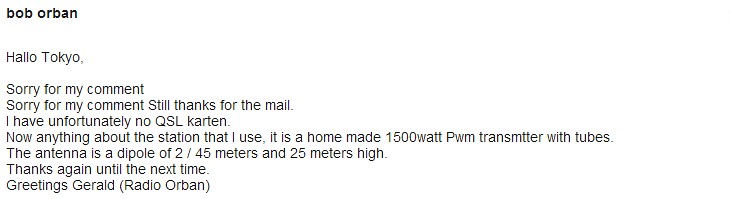The image is a clean, black-text-on-white-background screenshot, resembling an email or letter. In lowercase letters at the top left, it reads "bob orben." The message starts with "halo, tokyo," followed by "sorry for my comment. sorry for my comment, still thanks for the mail." The text continues with, "i have unfortunately no qsl carton. now, anything about the station that i use. it is a homemade 1500-watt pwm transmitter with tubes. the antenna is a dipole of 2, 45 meters and 25 meters high." It concludes with, "thanks again until the next time. greetings, gerald," followed by "(radio orban)."